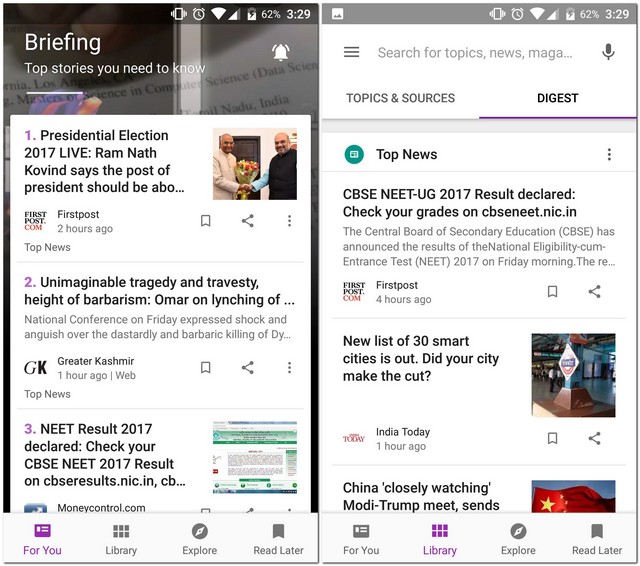This vertical image, typically found on a smart device, features two distinct sections. On the left side, the top part displays "Briefing" in white text, accompanied by the subtitle "Top stories you need to know." Above this title, various icons such as a clock, a filled triangle pointing sideways, a battery icon showing 62%, and the time "3:29" are visible. The background appears to be an image of someone reading, though it is heavily faded due to the overlay of multiple boxes and text.

To the right of the "Briefing" title, there's a bell icon. Below, a white box contains snippets of three different articles. The first article, titled "Presidential Election 2017 Live," features a picture and begins "Ram Nath Kovind says the post of the president should be about..." followed by an ellipsis. This article's details note it was published two hours ago and offers share icons for user interaction. The second article, "Unimaginable Tragedy and Travesty, Heart of Barbarism," is about Omar's comments on lynching, similarly providing specifics and share buttons. The third article states "NEET Result 2017 Declared, Check Your CBSE NEET 2017 Results" for readers interested in these results.

At the bottom, navigation options include "For You" (highlighted), "Library," "Explore," and "Read Later." Switching to the next page maintains the same header icons but changes the content. This page prompts users to "Search for new topics" and offers sections for "News" and "Magazines," with a microphone button for voice search and categories like "Topics" and "Sources." The "Digest" section is highlighted and underlined, showcasing top news articles with accompanying images. The bottom navigation mirror the previous section with options like "Top News," offering a consistent user experience across both pages.